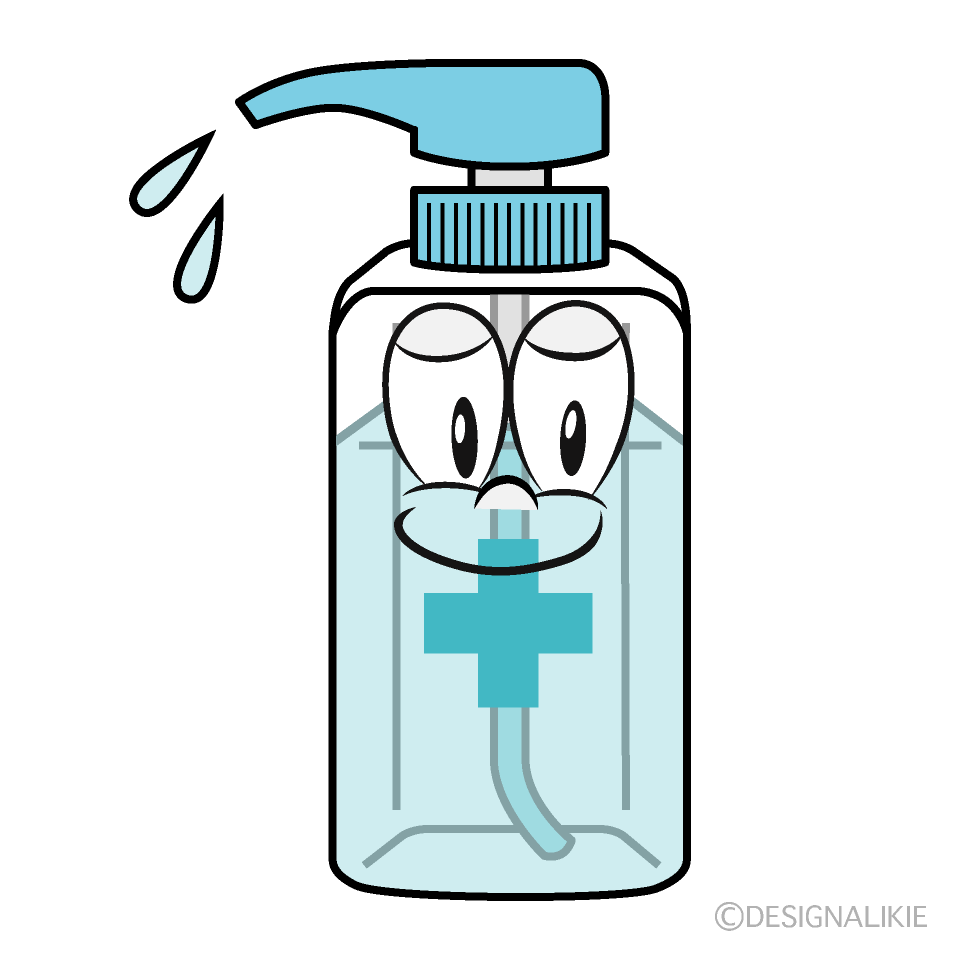This vertical rectangular image is a detailed and stylized cartoon drawing of a hand sanitizer bottle against a white background. The clear bottle contains a bluish liquid and features a blue cross symbol. A dispenser with a light blue tip and blue screw-on lid sits atop the bottle, with a gray tube running down into the liquid. Notably, the bottle is personified with a cheerful cartoon face, including two large eyes and a smiling mouth. Additionally, two graphic droplets are depicted near the dispenser. In the lower right corner, the text "© Design A Likey" is present, giving it a copyrighted and playful touch.